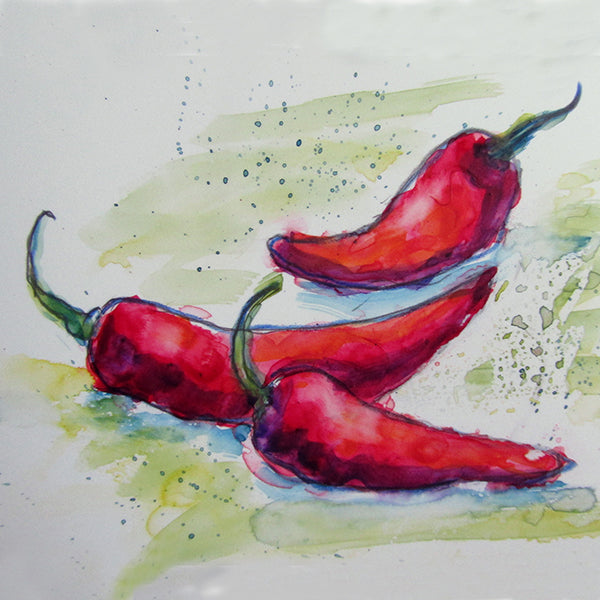This artwork is a simplistic, interpretive watercolor painting featuring three red chili peppers of varying sizes. The vibrant red peppers with green stems are arranged with one in the foreground, one in the middle, and one in the background, highlighting their differing proportions. The background is off-white, adorned with splatters and streaks of green and blue paint. The green streaks form a crescent shape underneath the peppers and continue partially on the right. Blue speckles are scattered throughout, some with a water-dried pattern indicating dried paint. The color application often extends beyond the outlines, giving the piece an abstract, expressive quality. Shadows of the peppers are rendered in blue, adding depth to the composition.